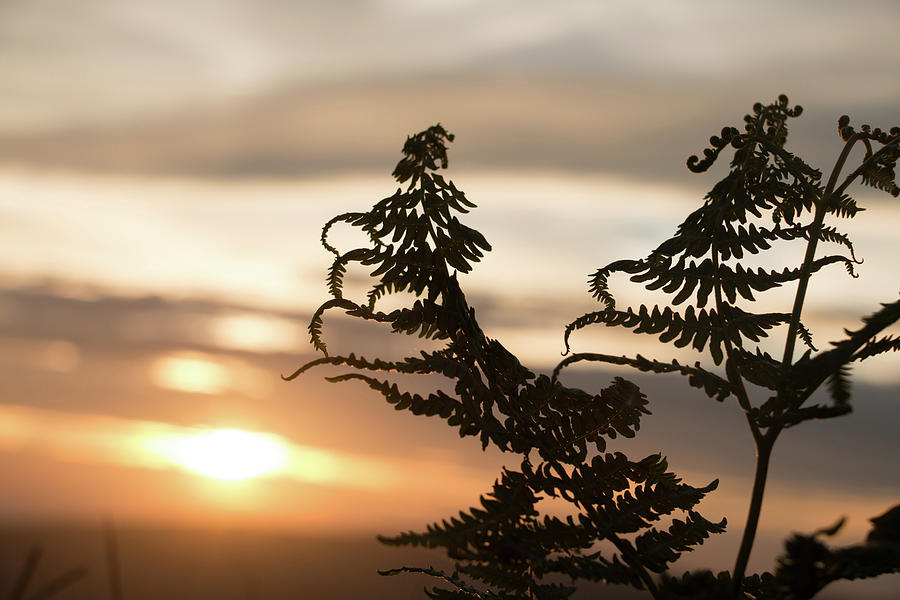The photograph captures a striking sunset scene, framed by two silhouetted fern stalks emerging from the right side of the image, with one extending towards the center. The delicate fern leaves curl gracefully to the left, their dark silhouettes contrasting starkly against the vibrant sky. The Sun, positioned in the bottom left, radiates through a nuanced palette that transitions from a bright white core to streaks of yellow, burnt orange, and dusky rose, finally blending into grayish-purple clouds with hints of blue. The background, filled with cloud patterns that streak across in layers, provides a blurred yet evocative setting that emphasizes the intricate details of the plant in the foreground. The entire scene exudes a serene blend of colors and forms, capturing the tranquil beauty of nature at dusk.